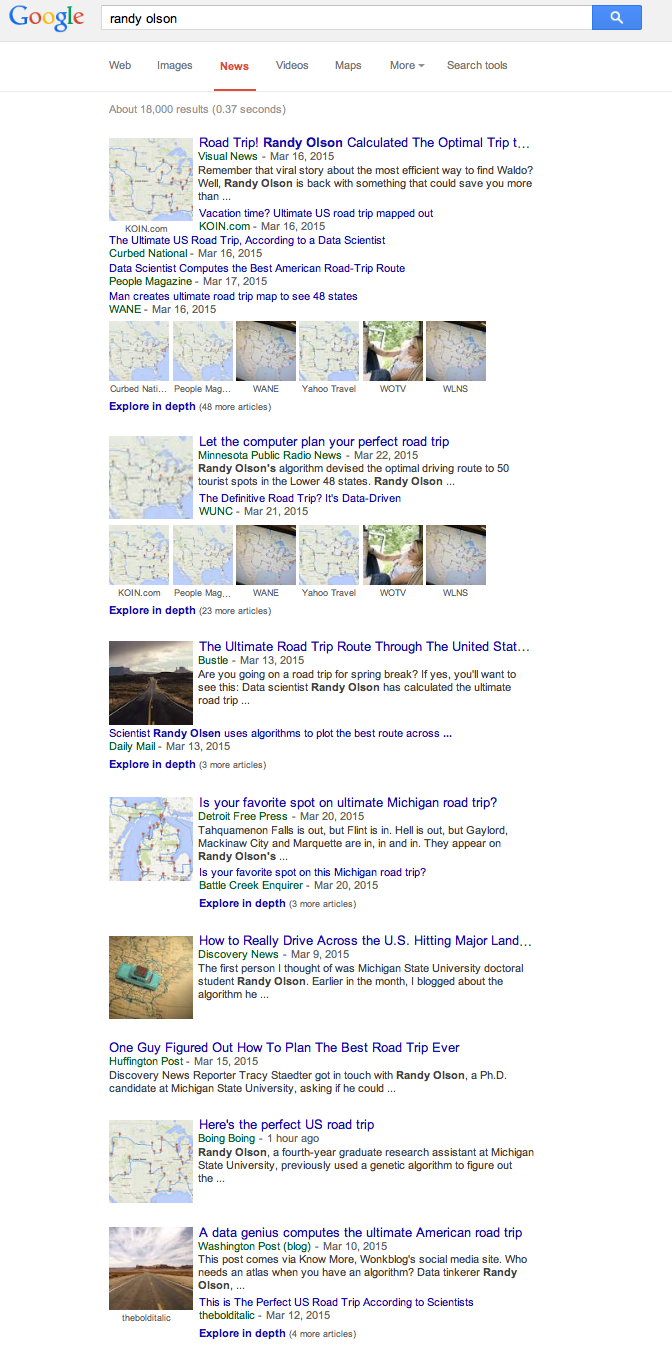This is a detailed, well-organized description of a Google search results page focused on "Randy Olson" and road trip planning content.

---

The tall, rectangular image displays a Google search results page. 

At the top left corner, the iconic Google logo is prominently featured, with its distinct colors: blue 'G', red 'O', yellow 'O', blue 'G', green 'L', and red 'E'. Directly to the right of the logo is a long search bar containing the typed text "Randy Olson" in black font. Located at the far right end of the search bar is a blue rectangle with a white search icon inside it.

Below the search bar is the menu, listing the search categories from left to right: Web, Images, News, Videos, Maps, More, and Search Tools. The "News" category is highlighted in red and underlined, indicating that it is the currently selected option.

Just beneath the menu, the page displays the search results, indicating that about 18,000 results were found in 0.37 seconds. 

The search results are organized in a column, each accompanied by images. The first result features an image that looks like a map, with the text "Road Trip Randy Olson" to the right, followed by additional descriptive text. Below this are six smaller images that appear to be various versions of maps. Underneath these images, the text "Explore in depth" is written in dark purple.

The next visual result includes a large map followed by six smaller images of different maps, one of which includes green elements. Below these images is a text snippet. 

The following row contains a photograph of a highway, seemingly taken from the perspective of a car driving along it with the sky in the background, suggesting an open road. To the right of the highway image, the text reads "The ultimate road trip through the United States..." with an ellipsis indicating more text to follow.

Further down, an image of a map of Michigan is displayed. To its right is a caption "Is your favorite spot on the ultimate Michigan road trip?" along with additional text. 

The next row includes a map with an image of a green and red car placed on it. The accompanying text states "How to really drive across the US, hitting major landmarks," followed by some more explanatory text. Below this row, a highlighted snippet reads "One guy figured out how to plan the best road trip ever" in purple, with "Huffington Post" in green beneath it.

Continuing down the page, another map is visible with the text "Here's the perfect US road trip" to its right.

The last row of results showcases another image of an open highway, set against a backdrop of sky and sprawling fields in shades of orange and brown. To the right of this image, the text reads "A data genius computes the ultimate American road trip," followed by more descriptive text.

---

This description provides a detailed and organized overview of the visual content and structure of the Google search results page displayed in the image.